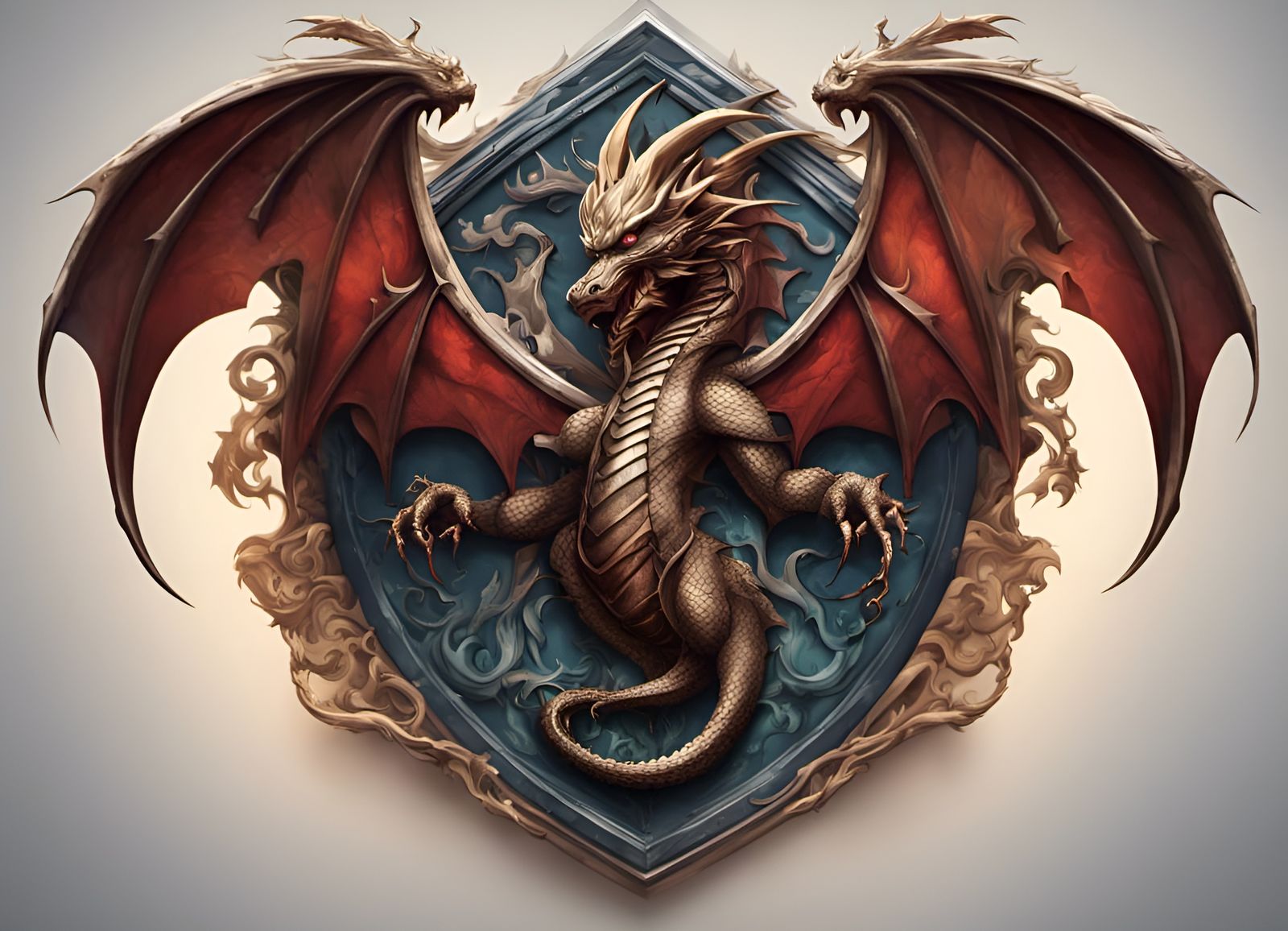The image depicts a highly detailed and playful animation drawing that evokes the aesthetics of Dungeons and Dragons or a video game. At its center is a blue, elliptical-shaped shield with a triangular top and pointed bottom, adorned with intricate beige or light-colored ornamentation resembling carved flames or vine-like claws. The border transitions from a light gray at the corners to an off-white or cream color toward the center. 

At the heart of the shield emerges a fierce, brassy bronze-colored dragon with red eyes and sharp spikes trailing down its head. Its wings, with red insides and brownish veins, stretch expansively beyond the shield, and its open mouth, clawed arms, and single curled tail contribute to a dynamic and menacing appearance. The entire composition, set against a plain and subtly colored background, gives the impression of a refined and fantastical crest or wall hanging, capturing the essence of heroic fantasy.